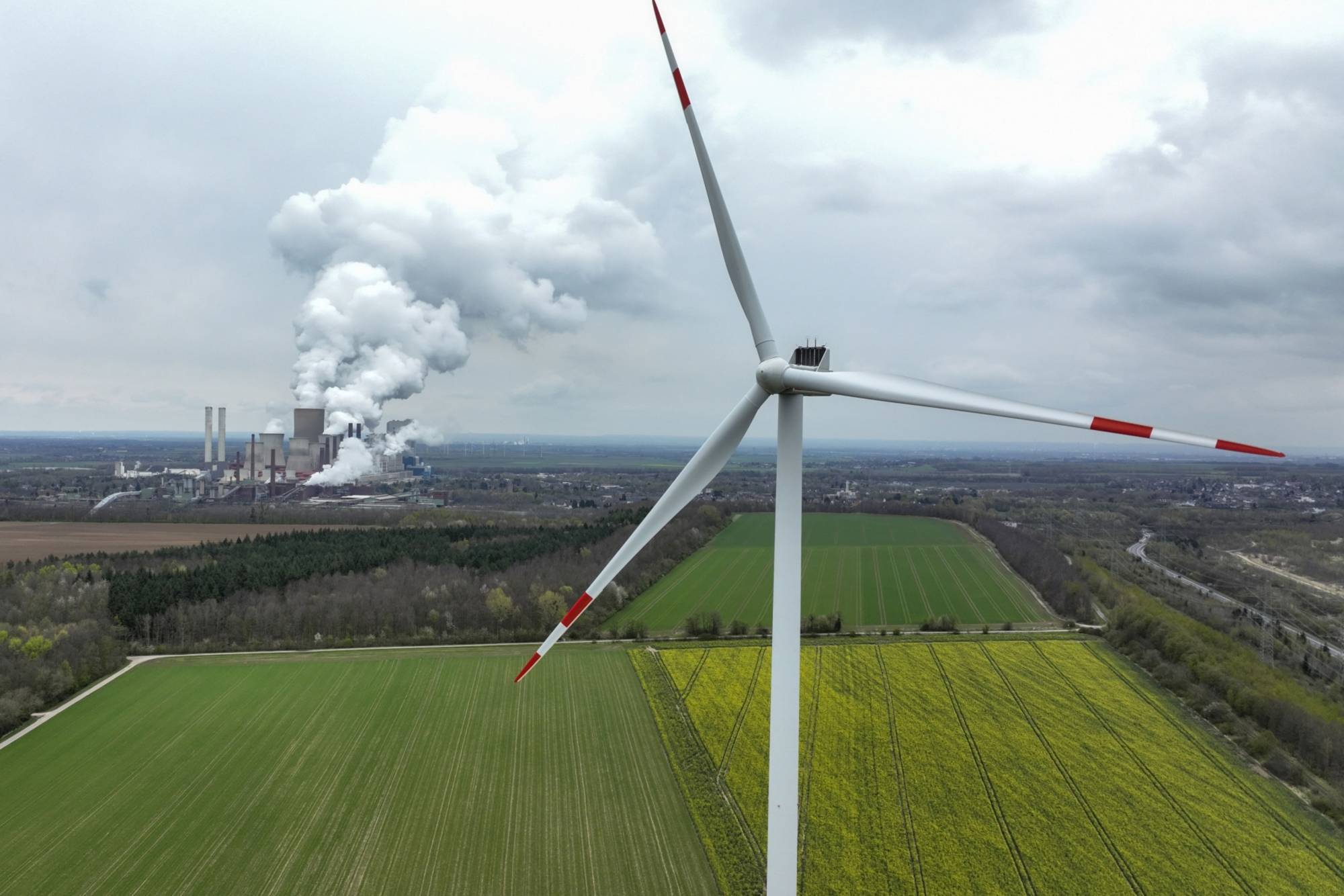The image captures an expansive outdoor scene dominated by a towering white wind turbine with three arms, each adorned with red and white stripes at the tips. The windmill stands prominently in the foreground, set against a backdrop of vast verdant fields, interspersed with a patch of yellow-green grass. On the left side of the horizon, an industrial area becomes visible, featuring several factories or plants characterized by large cement towers. These structures emit substantial plumes of white smoke that billow into the otherwise blue and partly cloudy sky. The scene is bathed in a soft, late afternoon light, accentuating the contrast between the vivid colors of the wind turbine and the surrounding natural and industrial elements.